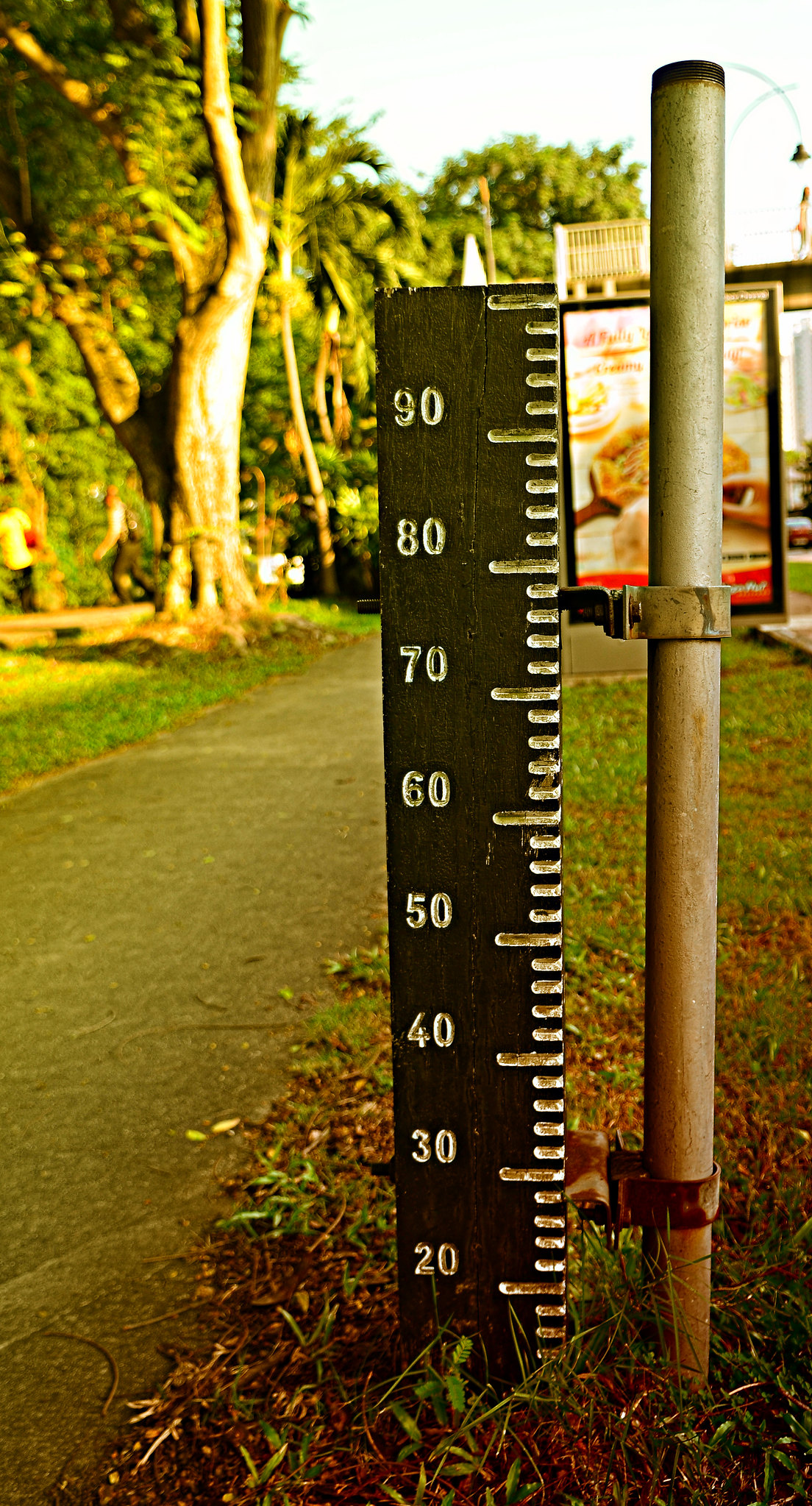In this image, we see an outdoor scene that appears to be a park or a natural field. Central to the composition is a large, black measuring device resembling a ruler, prominently mounted on a silver metal pole. The scale on this instrument ranges from 20 at the bottom to 90 at the top, with small ridges marking intervals in between. Its exact purpose is unclear—it could be a temperature gauge, a rain gauge, or some other measurement tool. The background reveals green trees and a brown grassy area intersected by a sidewalk. In the distance, a few indistinct figures can be glimpsed, though they are too far away to discern any details about them.